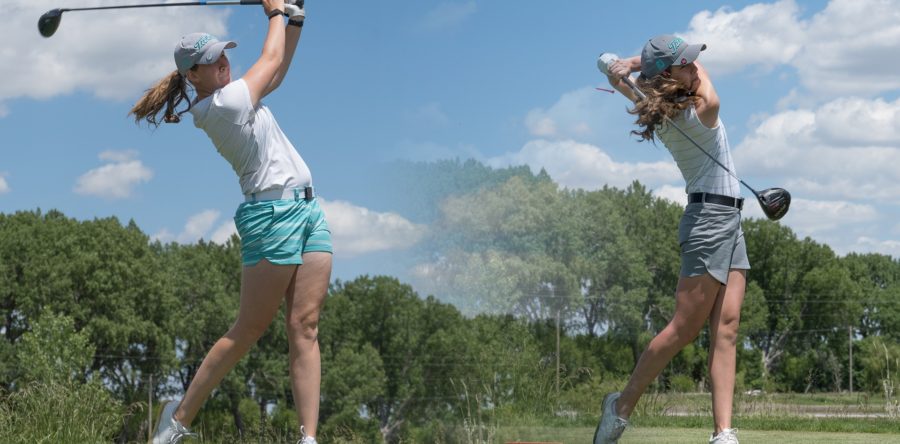The image depicts a dynamic and synchronized scene of two young blonde Caucasian women mid-swing on a golf course. The photo on the left shows a woman dressed in a white t-shirt and light blue shorts, her hair tied in a ponytail under a blue cap, and she's captured just after her swing, with the golf club high above her head. Her counterpart in the right photograph is wearing a white sleeveless t-shirt, gray shorts with a belt, and a darker blue cap. She has executed a powerful backswing, her club extended far behind her. Both women, sporting golf shoes, appear to be enjoying themselves on a lush, green driving range, surrounded by a beautiful landscape of rolling hills and green trees under a bright blue sky dotted with fluffy white clouds. The photographs are seamlessly merged with slight overlap, creating a coherent and energetic portrayal of their simultaneous swings.